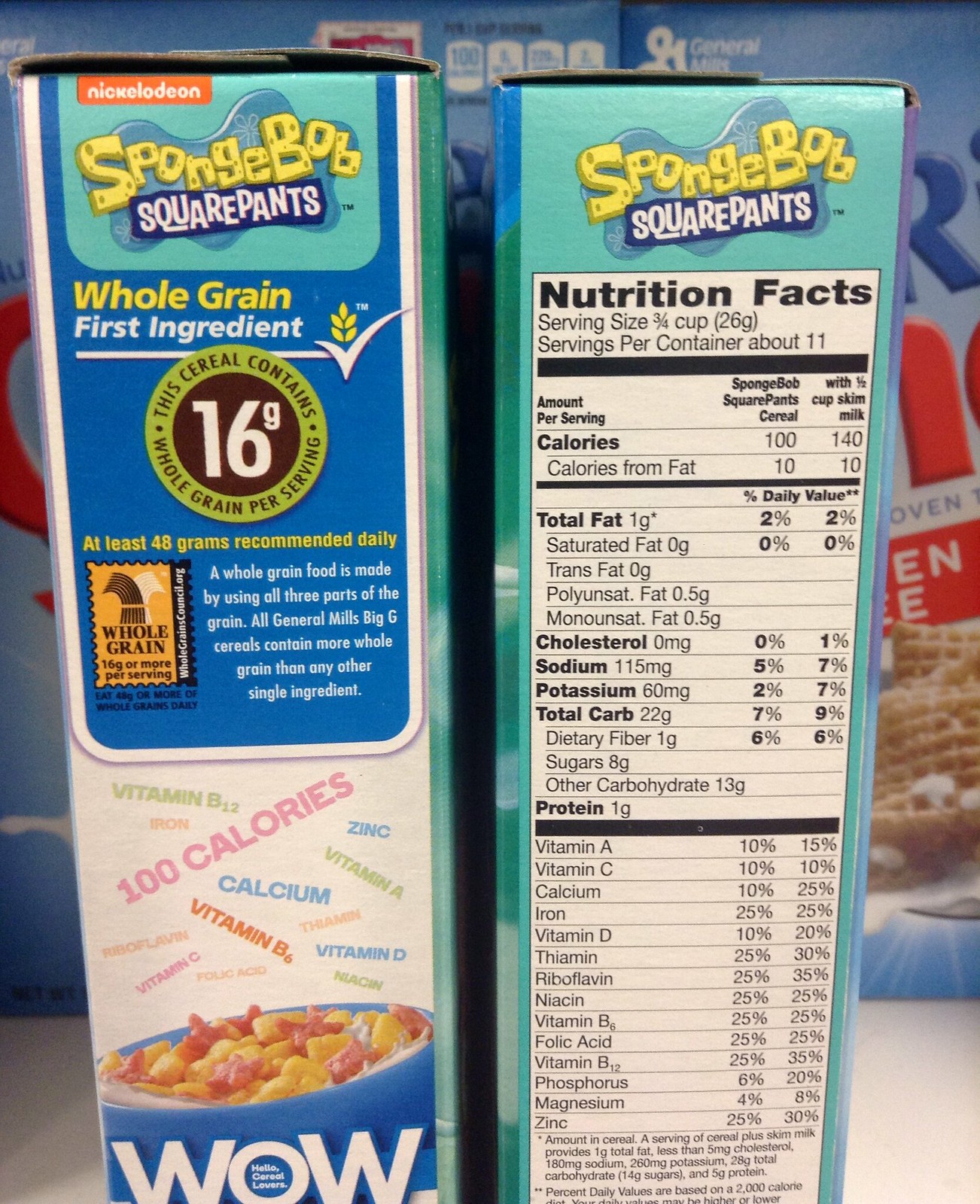This image features two cereal boxes prominently displayed side by side. On the left, there's a partial side view of a box, dominated by a light blue color along the edges. The central feature is a vertical blue rectangle that reads "SpongeBob SquarePants." Below it, text highlights "whole grain, first ingredient" in green-ish circles and mentions "16 grams" in brown with white print. Further down, a white section provides information about the cereal, accompanied by a picture of the cereal, and a bold "WOW" beneath it.

The adjoining box on the right shows another side of the same cereal, also branded with "SpongeBob SquarePants" at the top. This side features a white vertical rectangle with black nutritional information printed on it. Behind these two boxes, more cereal boxes are visible but mostly obscured, displaying a light blue color with hints of dark blue and red text. On the very right edge of the image, there's a small, enticing picture showing a bowl of grain-checkered cereal with milk.